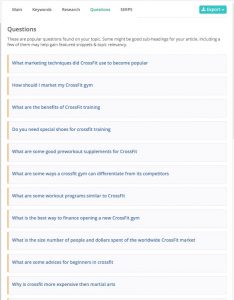The image features a white background with several blurry tabs and text. At the top-left corner, there are a total of five tabs; four of them are black, while the fourth tab from the left is green. Due to the blurriness, the words on these tabs are unreadable. On the top right, there's a green rectangle with white text, possibly labeled "export," but this is not certain.

Below this, there's a section labeled "Questions," possibly accompanied by a subtitle such as "These are popular questions about your topic," though the exact wording is unclear. Further down, two rows of beige rectangles with blue text can be seen, although the blurriness makes the text difficult to decipher. Some partially readable phrases include "What did ... become popular," "How should I ... my," and "What are the benefits of ...". Another phrase starts with "Do you," but the remaining words are indistinguishable.